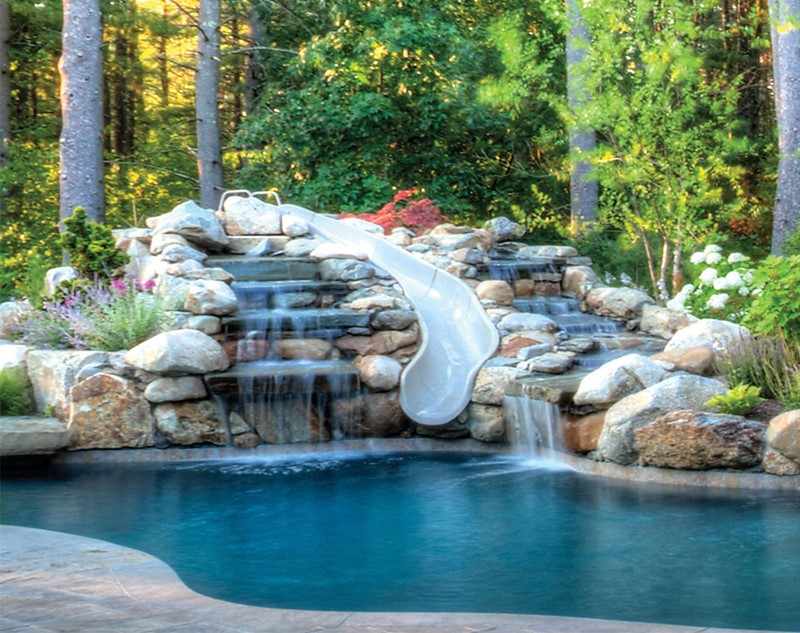This outdoor daytime photograph captures a stunning backyard swimming pool with an aqua blue hue at its center. Surrounding the pool is a tan deck at the bottom of the image closest to the camera. On the opposite side of the pool, a well-crafted water feature showcases a small tan water slide flanked by parts of a multi-tiered waterfall. This waterfall cascades down various levels of smooth light gray to white rocks interspersed with boulders. The water flows seamlessly, giving a polished, man-made appearance. Flowering plants and shrubs are strategically placed around the rocks, with light pink flowers emerging on the left and white flowers on the right, alongside a thin tree. Behind the water feature, a lush backdrop of trees, bushes, and vibrant green plants completes the scene, highlighting the natural yet artfully designed landscape.